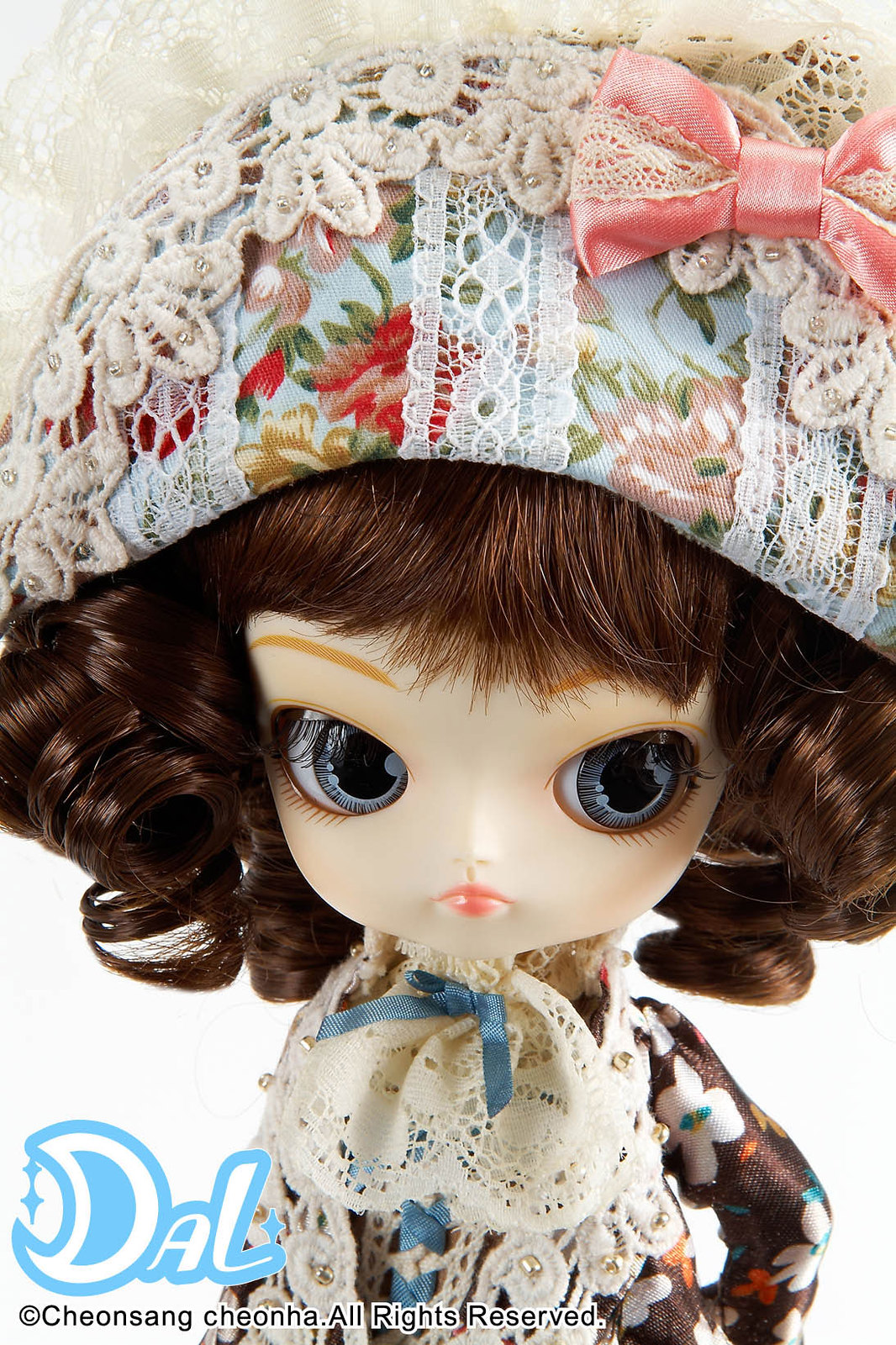This image depicts a striking D.A.L. doll that exhibits an intense expression. The doll is adorned with a large, elaborate hat made of a floral fabric and accentuated with white lace and a pink ribbon. Topping the sophisticated headgear, there is also a white fluffy hat reminiscent of early 1900s fashion. The doll's auburn hair is curly, styled with bangs that frame her unusually small head, while the sizable hat enhances the visual impact of her dark, auburn curls.

Her complexion is notably pale, contrasting with her big blue eyes, which dominate her face and contribute to a pouty or mean demeanor. Painted orange or brown eyebrows, a petite nose, and pink lips complete her delicate facial features. The doll's attire features a brown and white flower-patterned shirt embellished with lace. Around her neck, she wears a scarf or handkerchief tied with a blue ribbon, adding to her vintage, floral aesthetic. The doll's unusual proportions include a slender neck and thin arms.

Text in blue with a white outline on the left side reads "D.A.L.," and at the bottom left, it states, "Cheongsong Chinha All Rights Reserved." This suggests that the doll is likely of South Korean origin and is produced by Shion Sang.